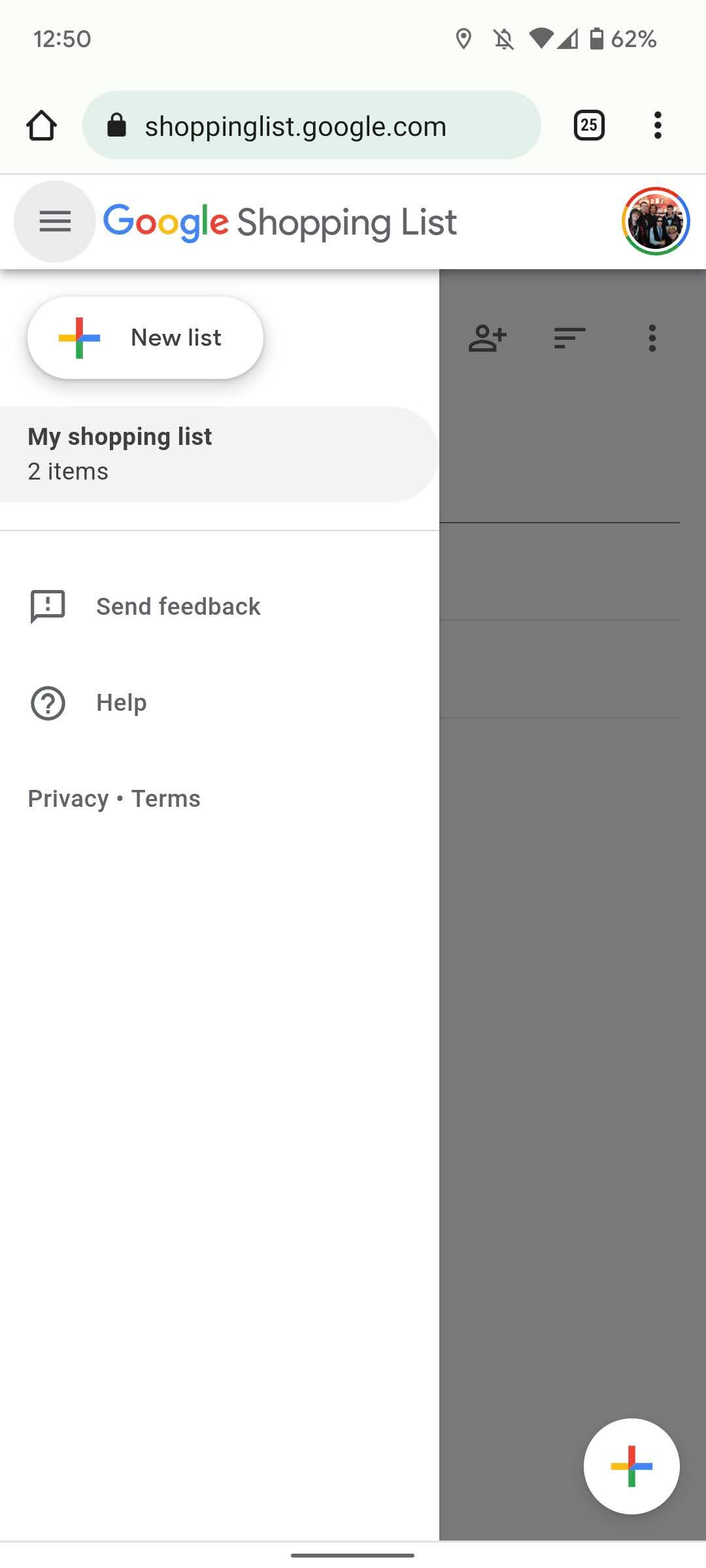On a mobile screenshot displaying the Google Shopping List interface, the main screen is predominantly occupied by an expanded left pane showcasing additional options. The background remains mostly blank, drawing focus on the interface details. At the top, "My Shopping List" is prominently displayed, indicating there are two items, although the items themselves are not visible. A minimalist design consistent with Google's aesthetic features a clean white background and dark text. 

A profile icon depicting a family indoors is located in the upper right corner, alongside a button labeled "New List." Another plus button appears in the bottom right, likely serving a similar purpose as the new list creation. The left pane also includes links for "Send Feedback" and "Help," along with privacy and terms links. Additionally, there is functionality to invite others to view the list, making it a collaborative tool.